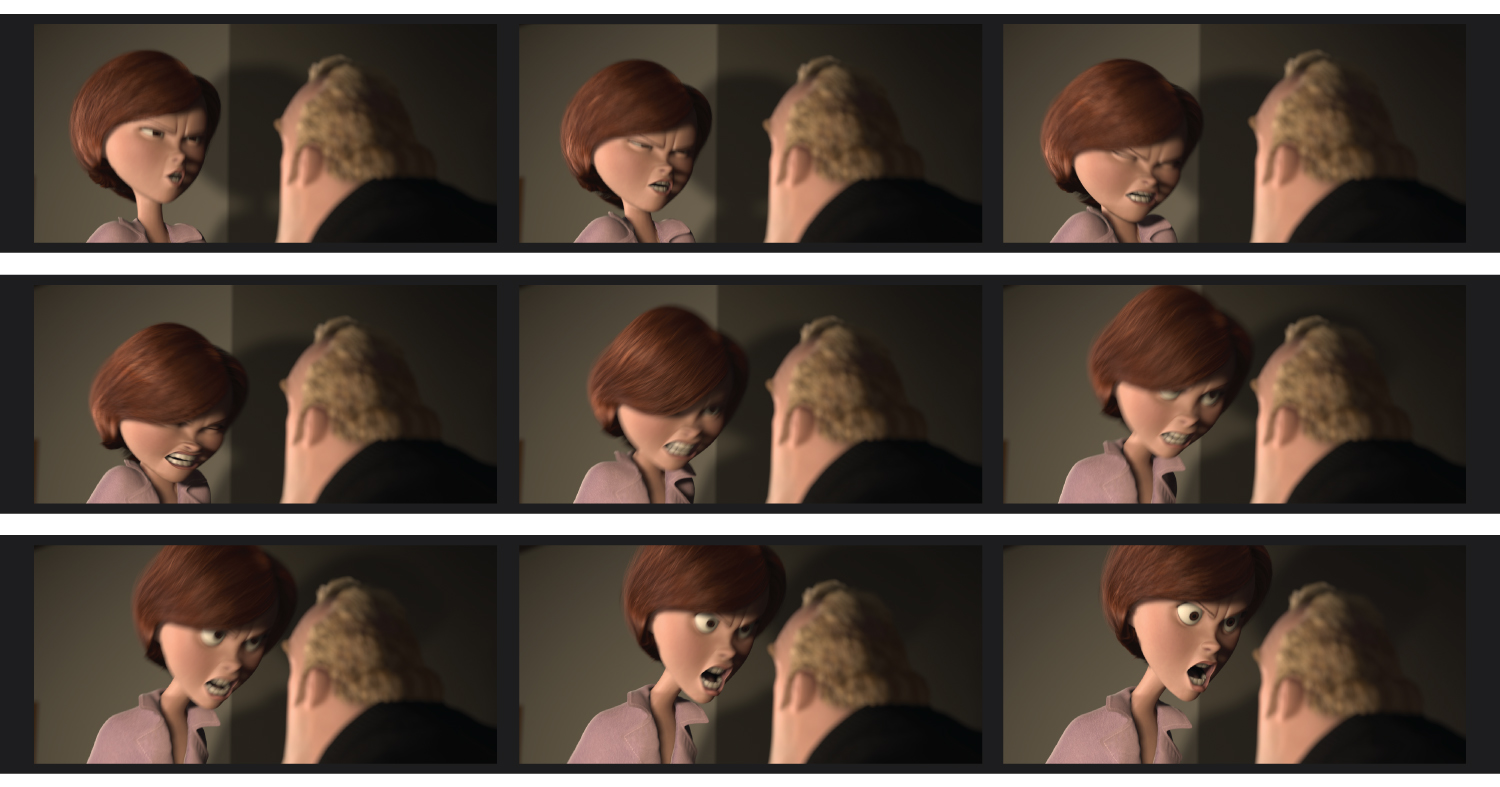A grid of nine sequential animated frames captures a scene reminiscent of Pixar's "The Incredibles." Each frame showcases a woman with short brown hair progressively displaying anger towards a man, who remains static with his back to the viewer. The man, characterized by his blondish hair and black jacket, does not move throughout the sequence. The artwork, comparable to styles from "Despicable Me" and "Toy Story," is vibrant and colorful. In the initial frames, the woman shows minor annoyance with a wrinkled nose. Her expression intensifies through subsequent frames: her eyes narrow, her nose scrunches up further, and her furrowed brow deepens. She eventually stands on her haunches, mouth open in a yell, confronting the man. She is dressed in a pink blouse with an open neckline. The detailed progression effectively depicts the gradual shift in her emotions, emphasizing the animation's focus on nuanced facial expressions.